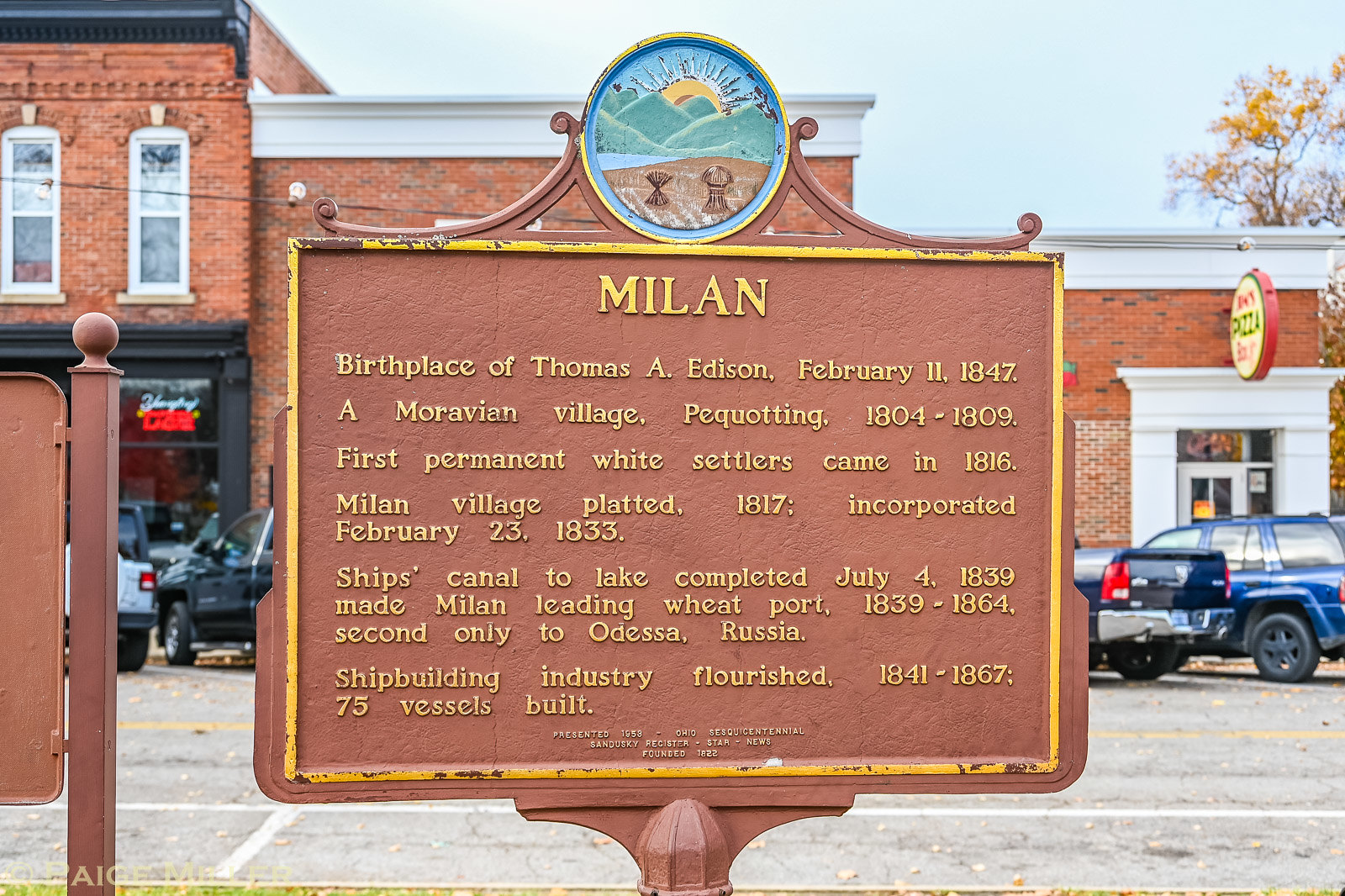The image features a street-side city plaque with a rough, orange-colored background and a yellow, peeling outline. At the top of the plaque is a circle with the shadowed silhouettes of green mountains, a sun, and a brown sea. The plaque reads, in yellow lettering: "Milan, birthplace of Thomas Edison, February 11, 1847, a Moravian village, Pequoting, 1804-1809. First permanent white settlers came in 1816. Milan village platted 1817, incorporated February 23, 1833. Ship's canal to lake completed July 4, 1839, made Milan leading wheat port, 1839-1864, second only to Odessa, Russia. Shipbuilding industry flourished 1841-1867, 75 vessels built." The background of the image showcases a row of red brick buildings with white details. The tallest building on the left has white-trimmed windows, while the middle building is partially obscured but identified as a pizzeria and possibly a bar. On the right stands the shortest building, featuring a door framed by a large white structure, with two vehicles parked in front—a blue SUV and a darker blue pickup truck. There are no people visible, just the buildings and parked cars.